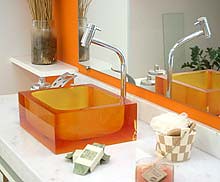The image showcases a luxurious bathroom setting centered on a pristine white marble sink adorned with subtle gray veining. The sink itself is designed in a sleek, square shape, resembling a modern box. A polished silver faucet arcs elegantly over the basin, with its tip directed downwards. Dominating the backdrop, a large mirror spans the wall, perfectly reflecting the sink and its surroundings. Upon closer inspection of the mirror's reflection, a hint of a lush green plant adds a touch of nature to the minimalist decor. Atop the marble countertop, an open package of soap, encased in green and white paper, is visibly situated. Additionally, there is a small, beige and white canister, likely containing a loofah or bath sponge, enhancing the sink area with functional aesthetics.